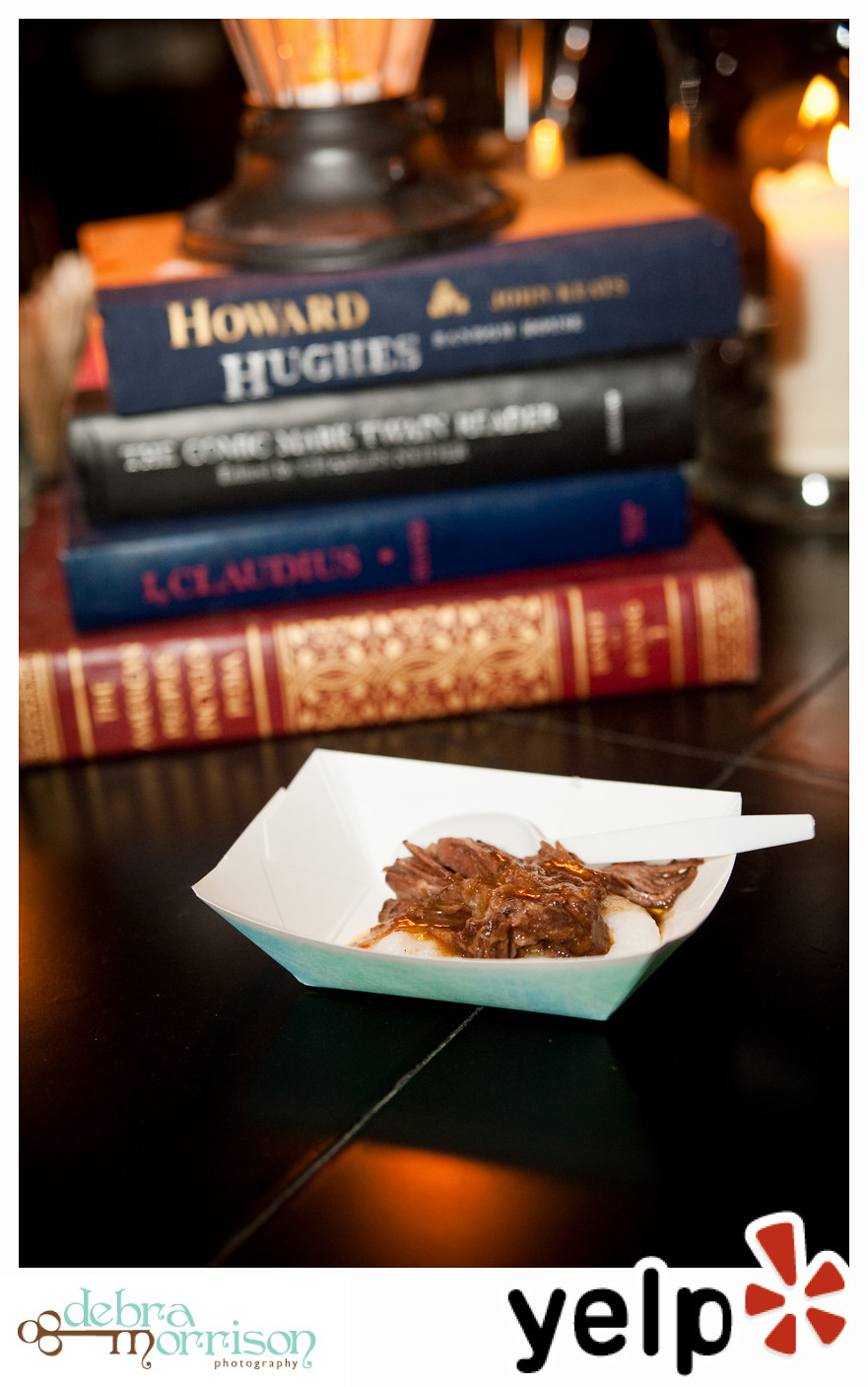This is an image sourced from Yelp, as indicated by the Yelp logo with red symbols in the bottom right corner. The photograph's credit goes to Deborah Morrison, whose name and logo appear at the bottom left. The focal point of the image is a white and blue tray, resembling a takeout container, filled with what looks like juicy shredded beef in gravy, sitting atop a bed of mashed potatoes. A white plastic spoon accompanies the meal. The setup rests on a black tabletop, with the background intentionally blurred to emphasize the food. Behind the tray, there's a stack of four books: prominently, a navy blue book titled "Howard Hughes," a black book with unreadable text, another navy blue book with pink writing, and a red book with gold lettering. On top of this book stack is a partially visible lantern. Additionally, a candle burns to the right, adding a warm glow to the scene.